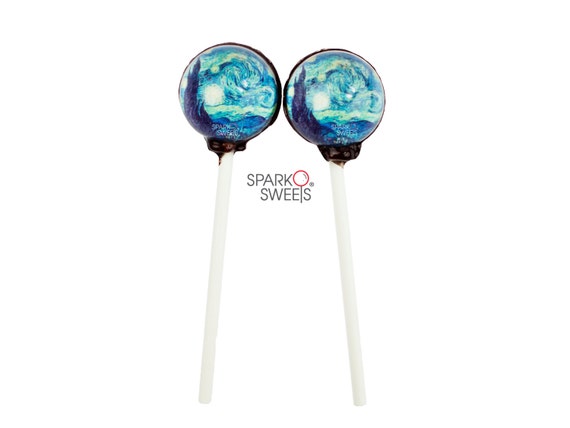In this portrait-oriented image, two upright and nearly touching suckers with white sticks are prominently displayed, each boasting a unique, iridescent blue hue resembling Van Gogh's "Starry Night." The spherical tops of the suckers are vibrant and eye-catching, creating an impression of lollipops. Nestled between the two sticks and positioned just below the candy portion, a logo in capitalized dark grey letters spells out "Spark O'Sweets." Notably, the "T" intersects the red "O" in "Sparko," giving it the appearance of a playful lollipop emblem.